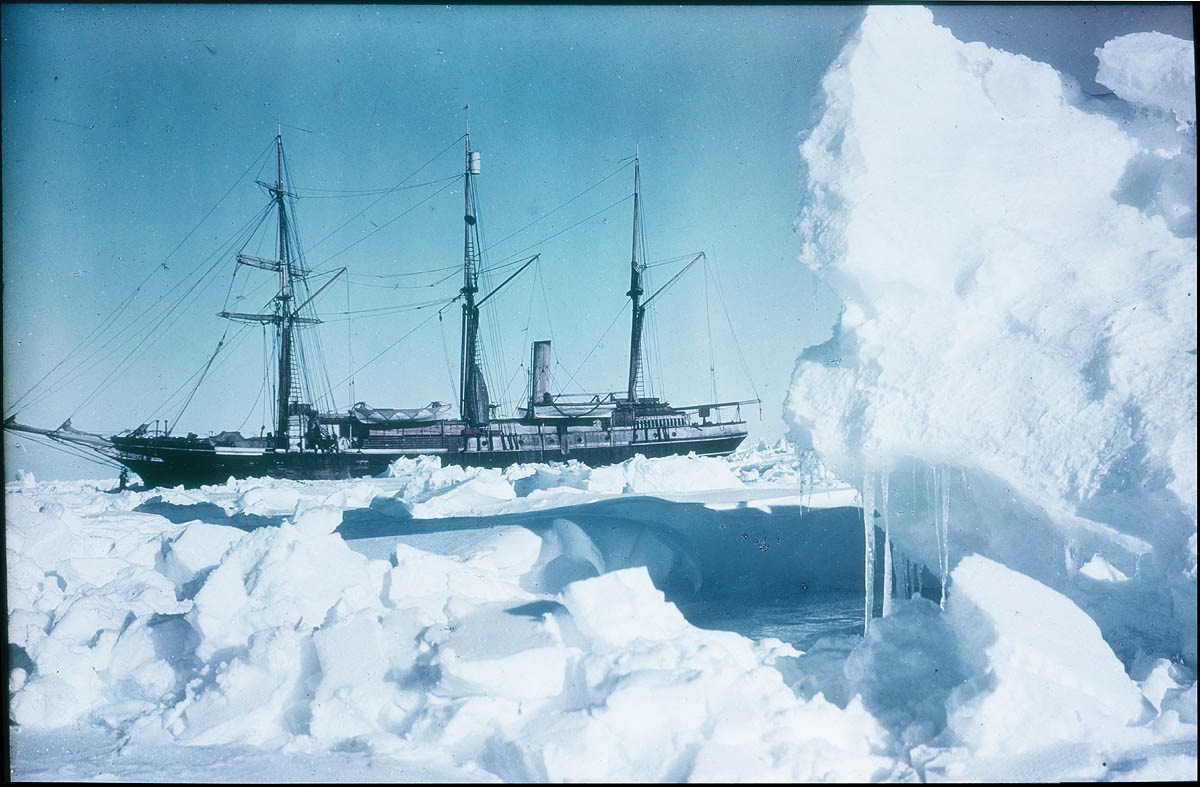The image is a rectangular wall art with a thin black border, depicting a large wooden ship, likely a fishing vessel, stranded amidst vast expanses of rugged, snow-covered ice, possibly in Antarctica. The ship, painted in dark browns and blacks, extends from the left to the right of the image. It features three vertical wooden masts with lines radiating in all directions for sails, though no sails are visible. The surrounding ice appears thick and jagged, with some chunks piled and shoveled to the lower left side, and a massive iceberg with dripping icicles sits on the far right. The background showcases a serene blue sky interspersed with white clouds, as the sun shines down, indicating it is daytime. The overall scene hints at isolation and the stark beauty of a frozen wilderness.